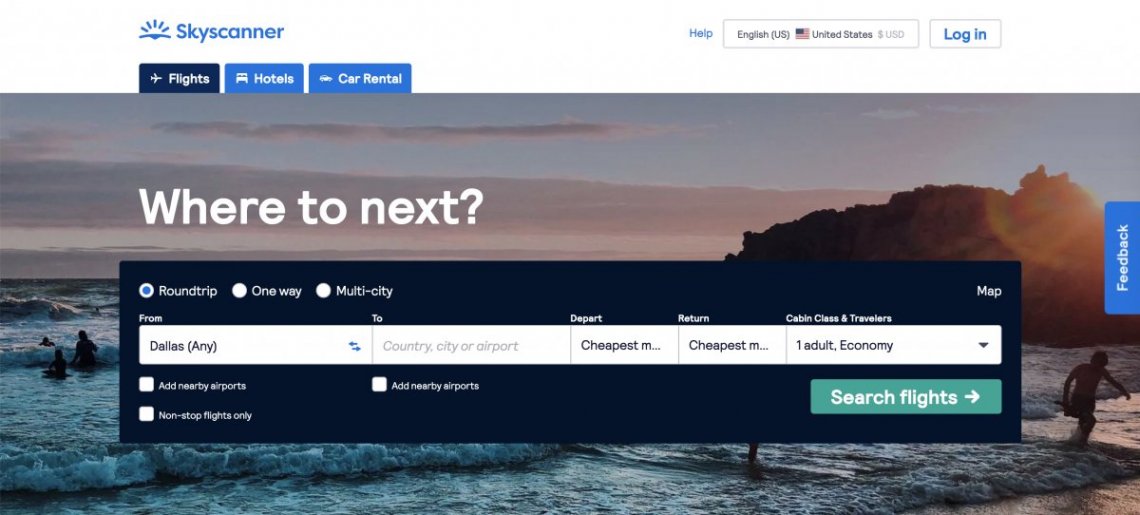The homepage of the Skyscanner website prominently features its distinctive logo on the upper left corner. The logo resembles a seagull flying directly toward the viewer with its wings extended, set against a backdrop of blue rays suggestive of a sunrise. To the right of this logo is a navigation bar with options such as "HELP," a search window currently displaying "English UK" and "United States," and a "login" button.

Below the navigation bar, there are buttons for "Flights," "Hotels," and "Car Rentals." The majority of the page is dominated by a visually striking image of an ocean scene, likely captured at sunset. The image features a few people in the water, backed by an array of pretty clouds with the sun setting towards the right side. Overlaying the sky in bold white lettering is the prompt, "Where to next?"

A pop-up box is readily accessible for users who wish to search for flights. This box allows users to choose between "Round Trip," "One Way," or "Multi-City" flight options, with the current selection on "Round Trip." The search fields include "Departure Location," "Destination," and other options. Additionally, the pop-up box highlights a selection for the "Cheapest" fare, set for one adult in economy class. The interface makes it easy for users to start their search for flights, aiding them in finding the best travel options.